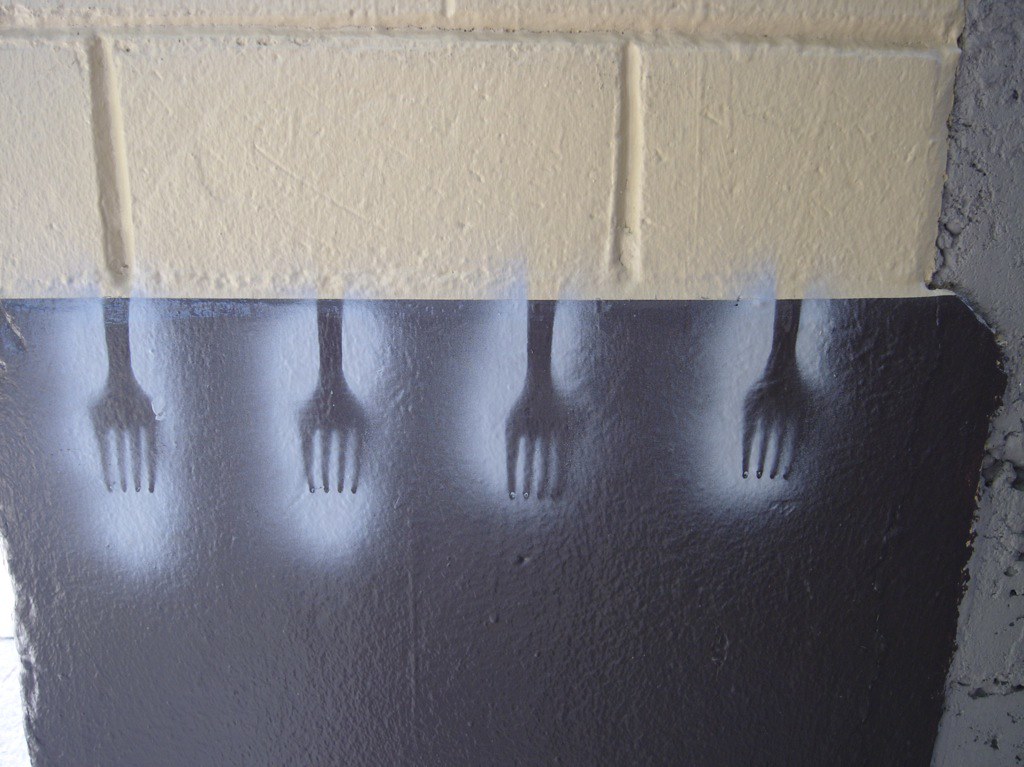This image depicts a wall that resembles a basement wall. The upper third of the wall is composed of cream-painted concrete blocks, while the right side features a section painted light gray. The lower two-thirds of the wall are more captivating; it's a single piece of cement predominantly spray-painted black. Four forks are stenciled onto this black portion, arranged horizontally with their prongs pointing downwards. These half-forks appear to glow with a bluish-white hue, creating an ethereal effect reminiscent of an X-ray or shadow art. Some overspray of this bluish-white paint marks the adjacent areas of the wall. The combination of stark black with glowing outlines gives the impression that the forks are mysteriously emerging from the wall. This unique visual is both intriguing and whimsical, as if it were an art installation one might find in an unconventional setting.